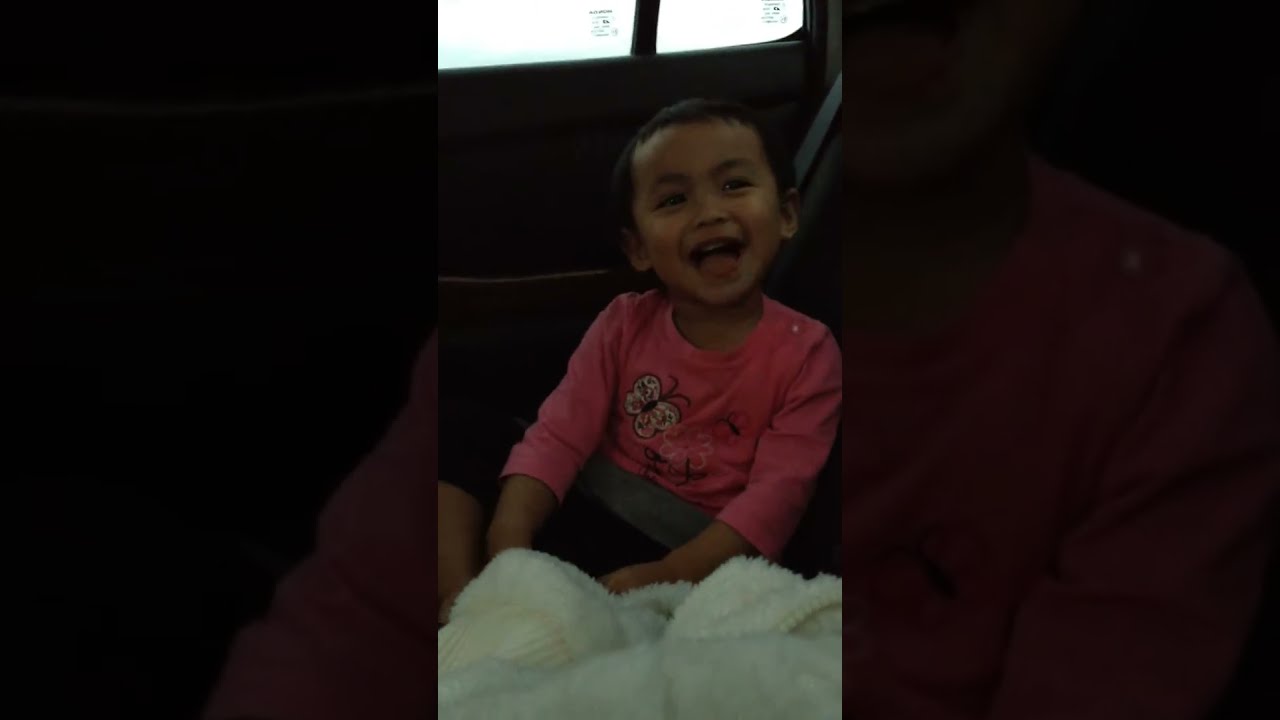A vividly joyful scene captures a young girl of likely Asian descent, happily seated and buckled in what appears to be a car seat, evidenced by the black seat behind her and the two vertical black strips on either side of the image. Her slightly brown skin glows with happiness as she beams with a wide smile, perhaps laughing in response to something amusing. She sports a pink long-sleeve or three-quarter sleeve shirt adorned with a playful design of butterflies and flowers in colors of white, pink, and black. This ensemble suggests she is enjoying a moment of carefree delight. Below her, a folded white jacket or blanket is visible, adding to the cozy scene. Her short dark hair frames her cheerful expression, which exudes natural, unforced joy. The image centers entirely on her, capturing an authentic and heartwarming moment.